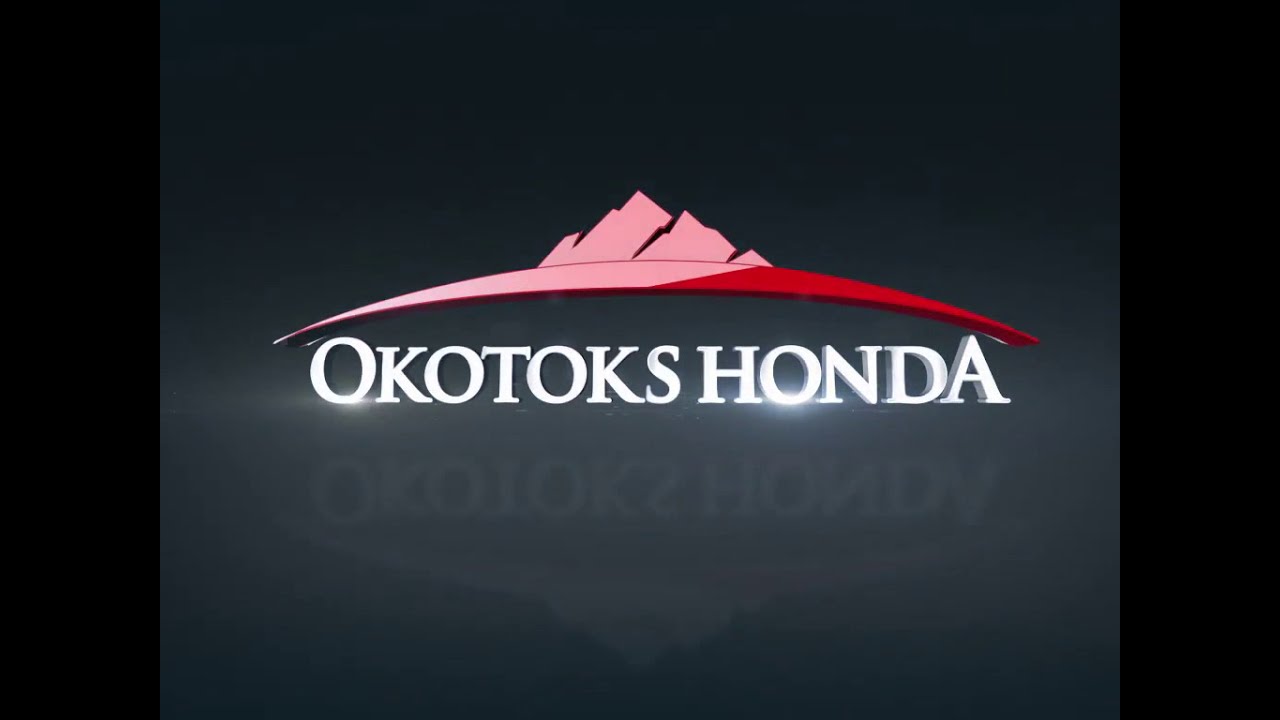The image is a promotional screenshot for a Honda dealership, specifically Okotoks Honda. The centerpiece of the image is the dealership's logo, which is prominently displayed and centered on a black background. This logo features a distinctive red arch or dome that stretches horizontally across the width of the text. At the apex of this arch are three stylized mountain peaks: one large peak with three jagged edges, a medium peak with two jagged edges, and a smaller peak resembling a pyramid. Notably, the arch is colored red on the right side and pink on the left side, creating a gradient effect. Directly below the arch, in bold 3D white text, is the name "Okotoks Honda," and this text is also centered. An interesting feature is the mirrored reflection of the logo and text beneath them, giving the impression that they are sitting on a reflective surface like water. The entire composition suggests a professional and visually appealing advertisement for the local Honda dealership.